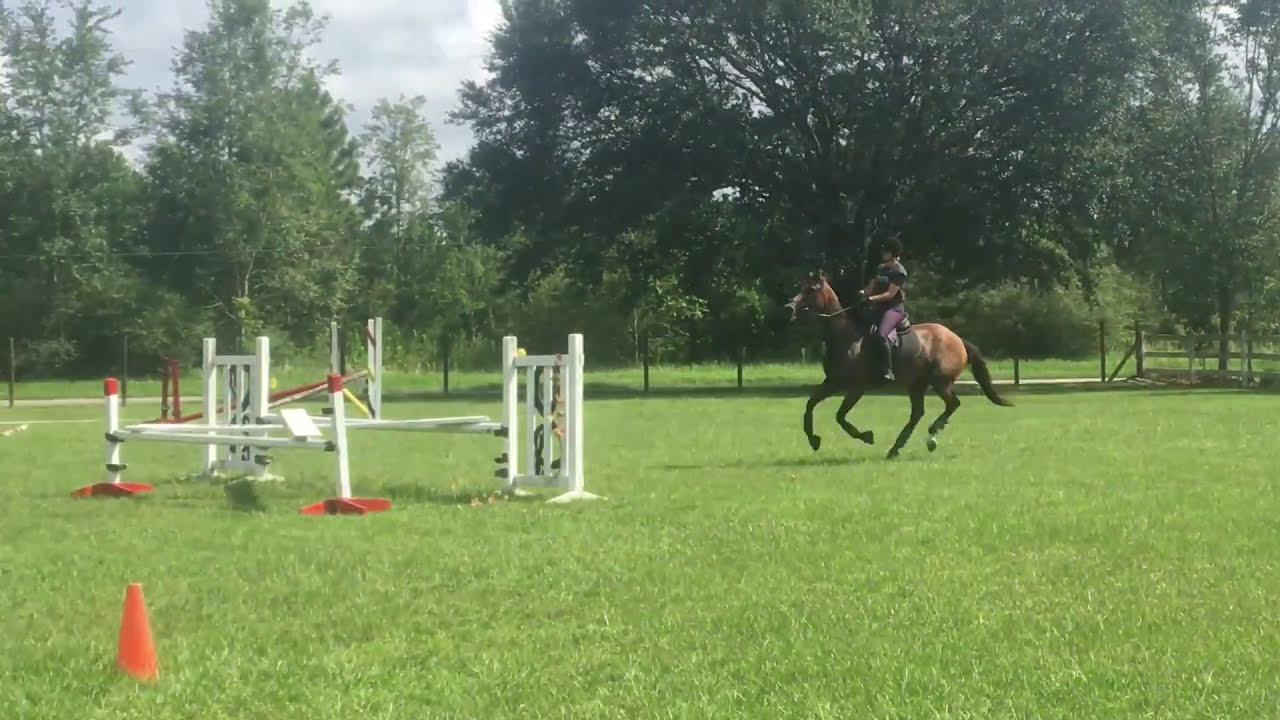In this outdoor image, a rider, possibly a woman, is seen riding a dark brown horse with a long black tail. The rider, clad in purple pants, white boots, and a black short-sleeved shirt, is on the right half of the scene, heading towards a set of hurdles on the left side. The hurdles are composed of white and red bars, with an orange column in the foreground. The horse is mid-stride, with three of its feet in the air and one on the ground, as they race across a field of green grass. In the background, there is a fence and an area that appears to be a gate, enclosed by trees and bushes. The scene is set on a sunny day with shadows of the horse and hurdles cast on the grass, and a blue sky with a few clouds peeking through the tree line, suggesting a pleasant, partly cloudy atmosphere. A couple of cones are noticeable near the bottom left corner, adding to the competitive setting of what seems to be a horse-riding event on a ranch.